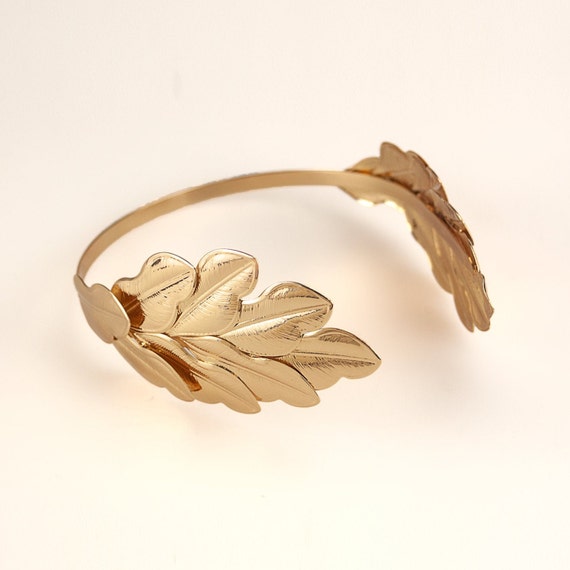The photograph features a gold-colored metal headband presented against a gradient background that transitions from a soft peachy-pink at the top to a nearly white hue in the lower right corner. The gold headband is thin and delicately curved, resembling the shape of an arch. Both sides of the band are adorned with intricate, embossed gold leaves, which have subtle flecks of brown near the tips and bases. This detailed and somewhat artificial presentation of the headband gives it the look of a product photo, such as one you might see on an e-commerce site like Amazon.